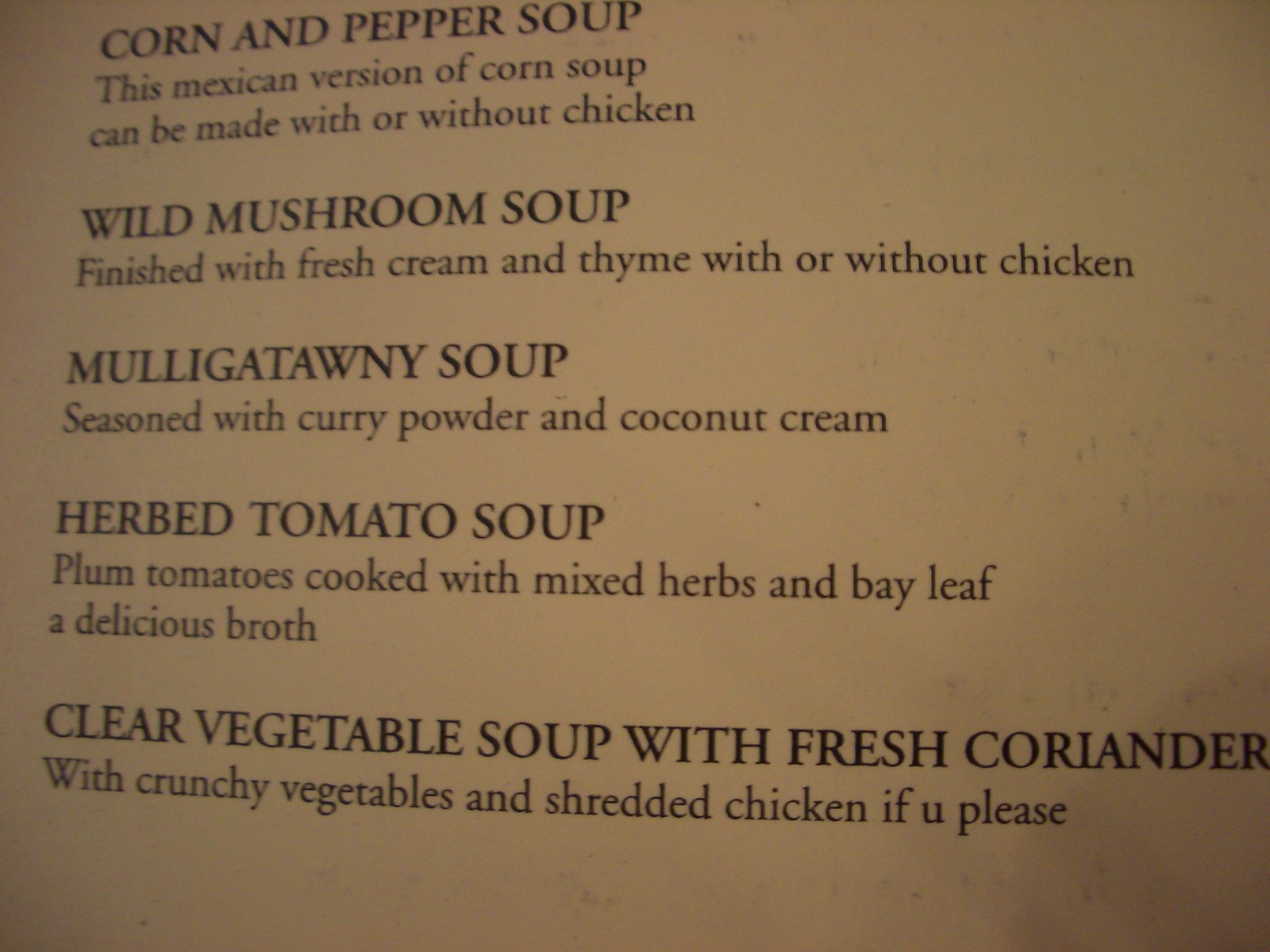The image depicts a cream-colored, possibly from a book or a menu, with black text detailing different types of soups. The titles of each soup are in a larger font than their descriptions, creating a clear hierarchy. The first item listed is "Corn and Pepper Soup," described as a Mexican variation of corn soup that can be made with or without chicken. Next is "Wild Mushroom Soup," which is finished with fresh cream and thyme and can also include chicken. Following that is "Mulligatawny Soup," seasoned with curry powder and coconut cream. The "Herbed Tomato Soup" features plum tomatoes cooked with mixed herbs and a bay leaf to create a delicious broth. Finally, there is "Clear Vegetable Soup," garnished with fresh coriander and crunchy vegetables, and optionally includes shredded chicken. The page appears to have a dim, yellowish-white hue, possibly due to lighting, with the text starting from the top left corner and aligned horizontally down the page.